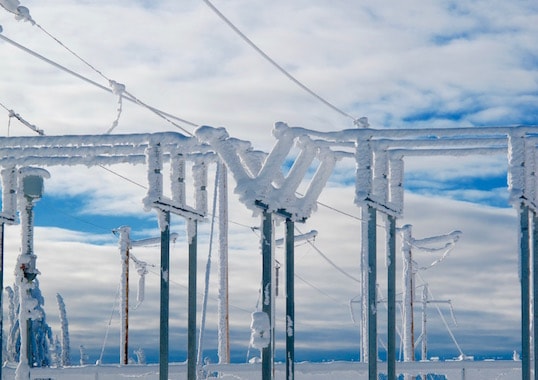The photograph displays an array of power lines and electrical poles, all coated in a thick layer of white frost, giving the impression of white poles. These structures, leading off into the distance, are enveloped in frost so dense it appears as though a thick coat of ice has formed over them. The scene is set against a vivid blue sky, filled with an abundance of fluffy white clouds, adding to the striking contrast against the frosted electrical framework. The image highlights the stark transformation of normally dark poles into impressive icy specters against a dramatic sky.